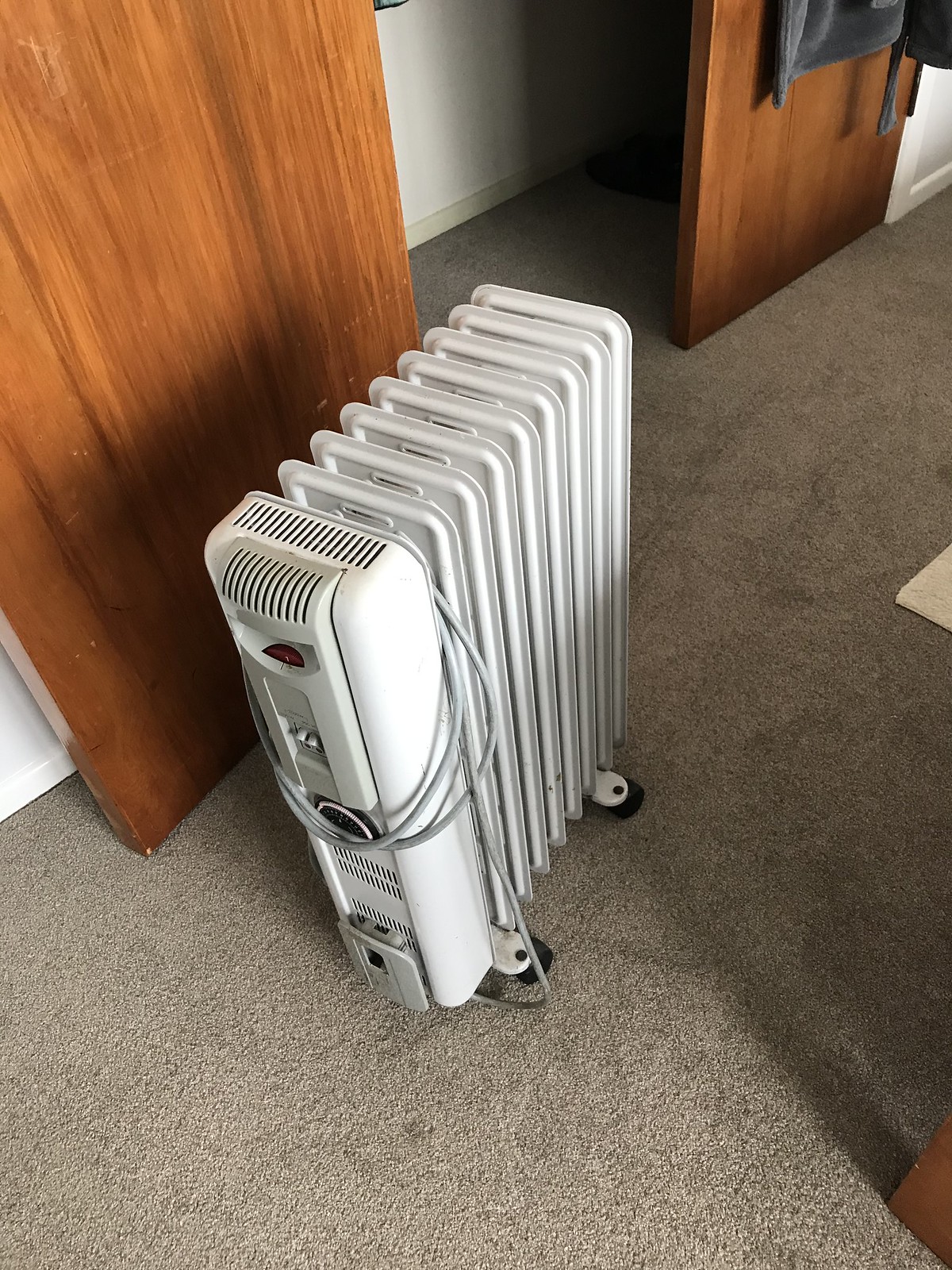This indoor photograph, lit by natural lighting, captures a white metal radiator-style space heater situated on a grey carpet, which may appear beige under certain lighting. The heater, featuring radiator coils and front vents with buttons, is equipped with wheels and an extension cord wrapped around its right side. It sits in front of a closet with brown wooden doors, one open and one closed, with an item, possibly a bathrobe, hanging on the outside of the closed door. In the background, there seem to be storage areas, likely the closet, and a faint glimpse of something hanging inside it. Additionally, part of a rug is visible on top of the carpet, along with the corner of another piece of furniture in the bottom right-hand corner of the image.